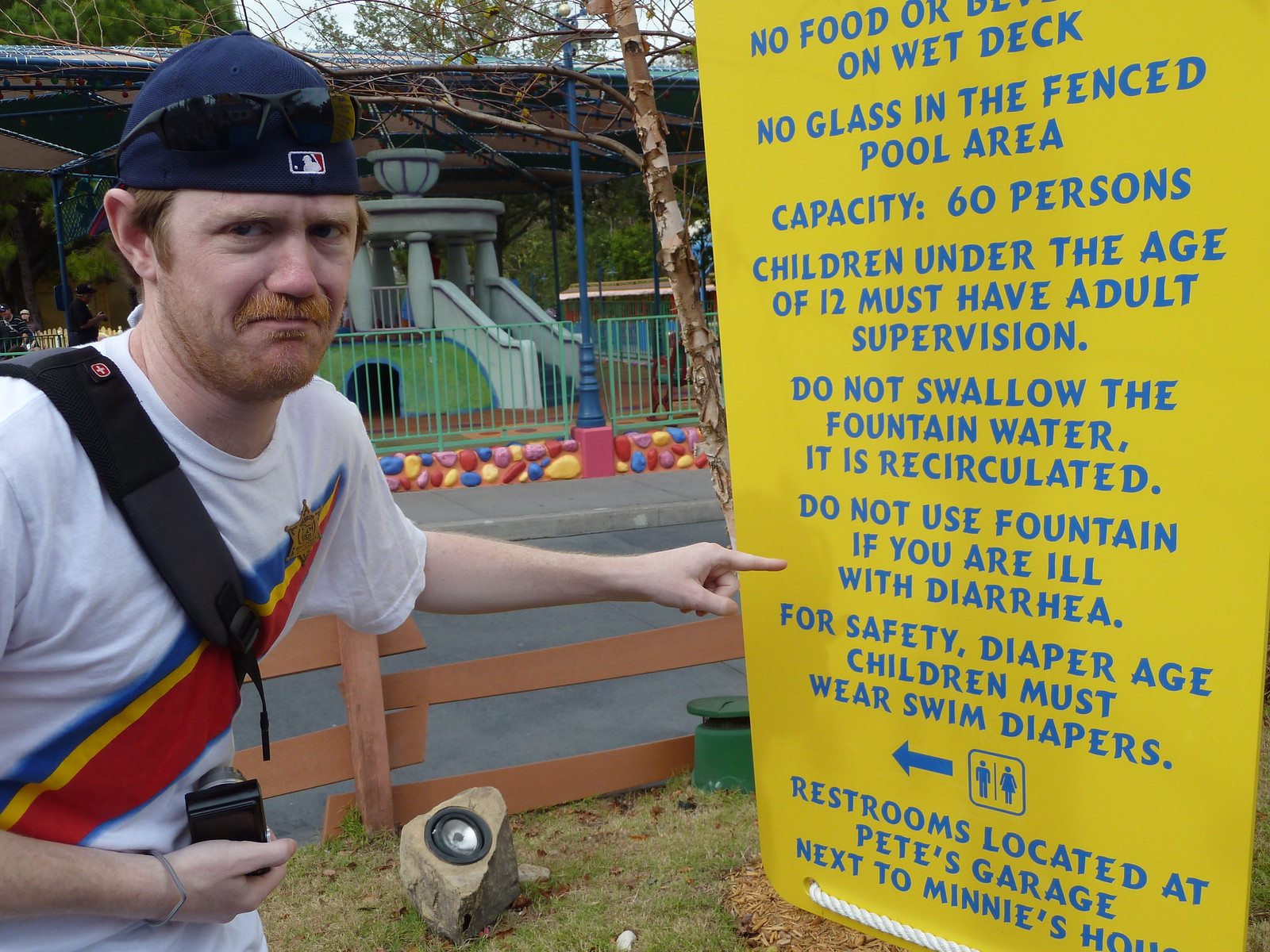This is an outdoor daylight color photograph of a man with fair skin and red hair, wearing a blue baseball cap backwards with a small red, white, and blue MLB logo on the front. He has sunglasses perched atop the cap. The man sports a mustache and a bit of stubble on his chin, and he's dressed in a white t-shirt with a blue, gold, and red slash across it. A black strap from a book bag loops over his shoulder while he holds a digital camera in his right hand. With his left hand, he points at a tall, upright, bright yellow sign with blue text. He has an unhappy expression, slightly holding his tummy as he points at the portion of the sign that reads "Do not use fountain if you are ill with diarrhea." The sign also includes various other notices such as: "No food or something on wet deck," "No glass in the fenced pool area," "Capacity 60 persons," "Children under the age of 12 must have adult supervision," "Do not swallow the fountain water. It is recirculated," and "For safety, diaper age children must wear swim diapers." Additionally, there is an arrow with symbols for men and women's bathrooms and a note that says, "Restrooms located at Pete's Garage next to Minnie's house." Behind the man and to the left, there is a grassy area with a rock that has a light fixture and a stone fence. Further back, beyond a green metal railing, there is a sidewalk, a street, and several buildings including some with canopies and green trees rising in the background.